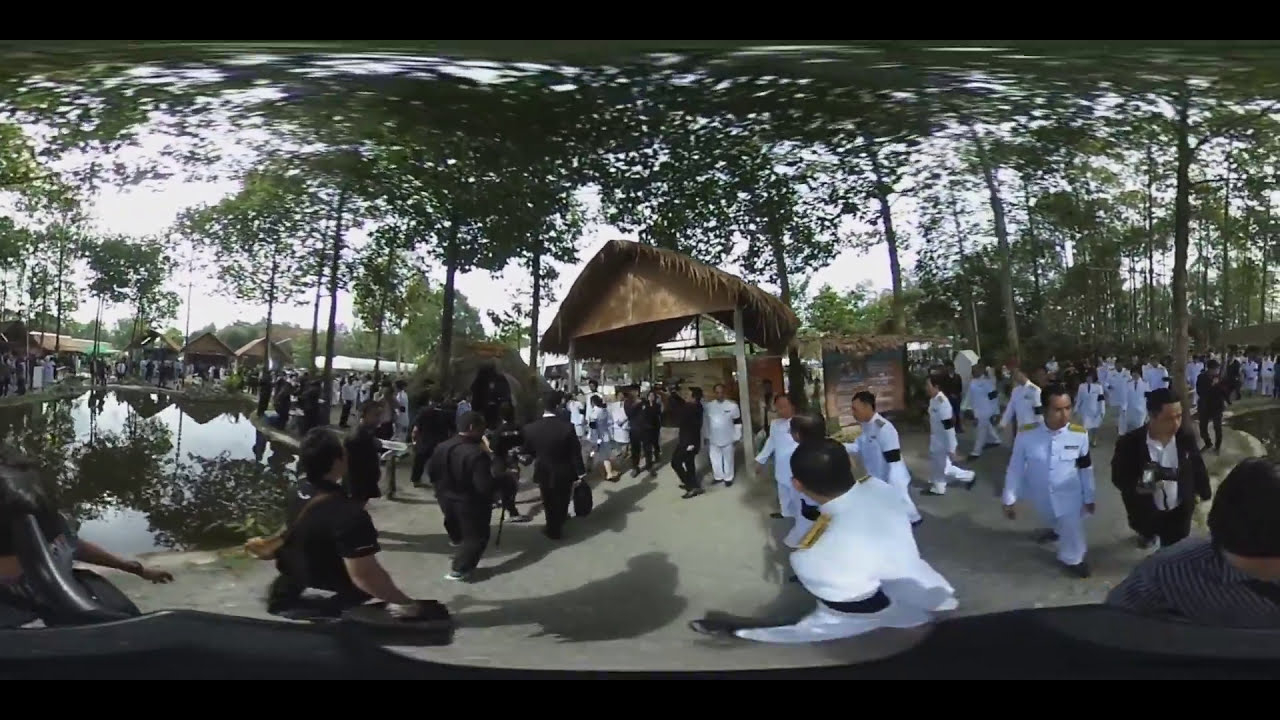This horizontally aligned rectangular image captures an outdoor scene during the daytime. The upper portion of the photograph features tall, narrow-trunk trees with abundant green leaves, juxtaposed against a bright, almost white sky, possibly due to a blur or 360 stitching effect. The trees appear slightly curved towards the viewer, enhancing the distorted perspective.

At ground level, a grayish surface, likely dirt or concrete, supports a bustling scene primarily populated by people in uniform. On the right, there is a group of individuals dressed in white military uniforms with yellow shoulder insignia and black bands wrapped around their left elbows. These individuals appear to be predominantly Asian with short black hair.

The left side of the image showcases another group of men dressed entirely in black, carrying what seems to be suitcases or bags. This group walks toward a prominent open hut structure with a brown roof supported by four posts, under which more people—some in black and some in white—are gathered.

Additionally, a small pond on the left side reflects the surrounding trees and adjacent grassy huts that extend into the background, amplifying the natural setting. Overall, the dynamic composition, diverse uniforms, surrounding trees, and water elements suggest a vibrant, possibly ceremonial gathering in a serene, small-town outdoor environment. The image does not contain any visible text.